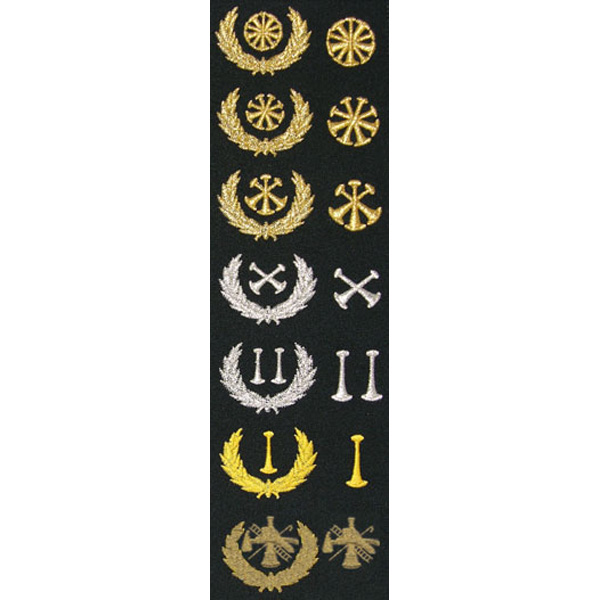The image displays a rectangular black fabric with 12 distinct, embroidered military-style patches arranged in two vertical columns. Each column contains six patches. The left column features golden laurel leaves beneath each patch, whereas the right column consists solely of the emblematic designs without laurel leaves.

At the top left, the first patch is a gold circle with eight spokes, resembling a wheel with crossed candlesticks inside. Directly below, the second patch showcases a golden wreath with a similar spoke design. The third patch follows with three crossed spokes, adorned with the same golden wreath. The fourth patch features silver wings crossed by two spokes, accompanied by a wreath. The fifth patch depicts silver wings and vertically placed spokes, again with a wreath below. The sixth patch displays various tools—an axe, ladder, and hook—crossed over each other within a brown wreath.

On the right side, the patches are identical in sequence and design to those on the left, minus the golden wreaths. As a result, the right column begins with the eight-spoked circle, followed by six spokes, then three crossed spokes, followed by silver wings with crossed spokes, then silver wings with vertically placed spokes, and finally, the tools crossed without the additional wreath. This intricate arrangement underscores the diversity and precision of military insignia.